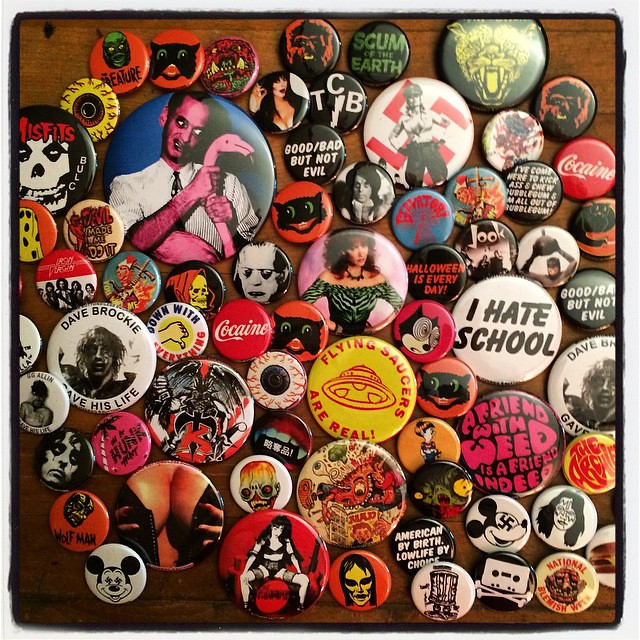The photograph showcases a vibrant collection of approximately 30 to 40 vintage pins, meticulously arranged on a wooden surface. These pins, popular in the 1980s, are intended for adorning jean jackets, sweaters, and other clothing. The pins display a wide range of colorful designs and slogans, reflecting a diverse array of themes from pop culture to humor. Among the notable pins are an Elvira, Mistress of the Dark pin; a Misfits pin featuring a skeleton head; a "Cocaine" pin styled like the Coca-Cola logo; and a pin proclaiming "Flying Saucers Are Real." Other pins include images of Mickey Mouse from different angles, slogans like "I Hate School" and "A Friend with Weed is a Friend Indeed," and portraits of figures such as Peggy Bundy and potentially John Waters. The collection also includes various animal heads, cartoon characters, and a controversial Nazi symbol. They range in size and imagery, featuring both colorful and monochromatic designs. This eclectic mix of pins, with their striking visuals and playful messages, provides a nostalgic glimpse into the quirky and rebellious spirit of past decades.